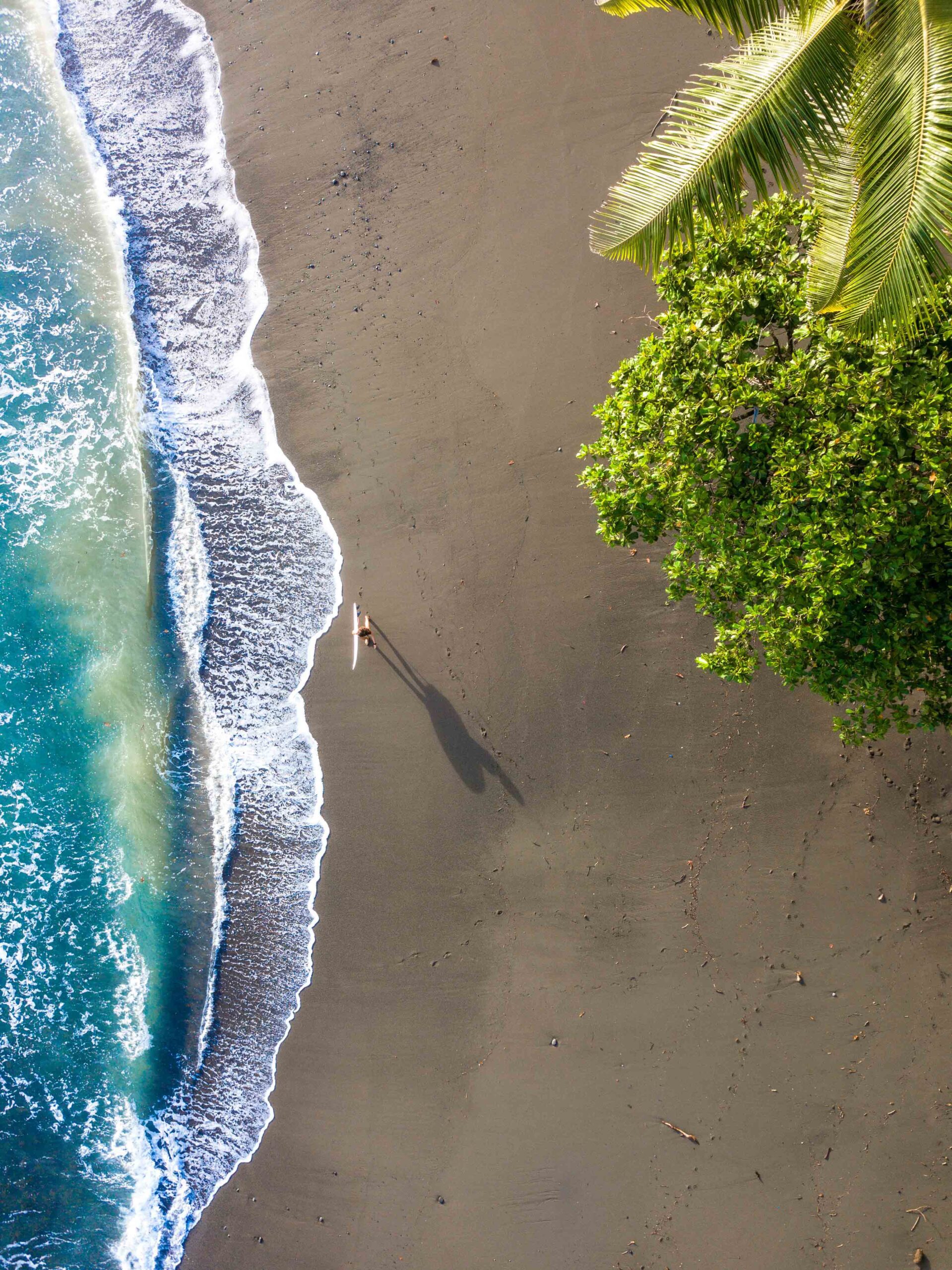This overhead, bird's-eye view captures a serene beach scene during the late afternoon. The image features a surfer walking along the dark tan sandy beach, holding a white surfboard, with their shadow slanting to the side, indicating the time of day. To the left, gentle waves roll in, creating a scalloped pattern of white foam against the bright blue water, which fades into green and teal hues. The beach appears largely clean, with subtle tracks visible in the sand. In the top right corner, the lush fronds of a palm tree and the verdant leaves of another tree add a touch of greenery to the coastal landscape.